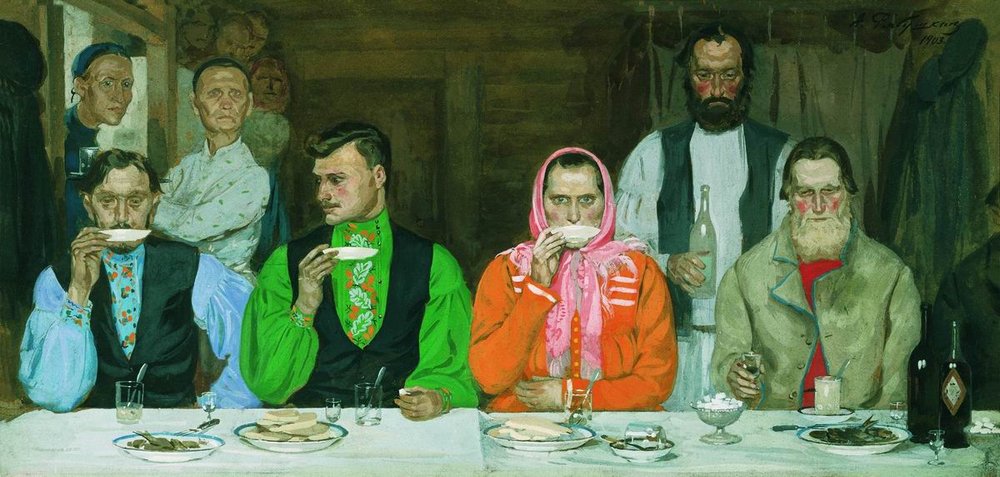This colorful, modern painting depicts a dinner scene set in a rustic cabin or barn. A long rectangular table covered with a white tablecloth occupies the lower portion of the painting. The table is laden with various communal dishes, two bottles on the right, and empty glasses each containing a spoon. Four individuals are seated around the table, facing the viewer. 

On the left, a man with darker skin, black hair, and a mustache, is wearing a blue shirt and black vest, holding a plate to his lips with his right hand. Beside him is a younger man in a green shirt and black vest, also holding a plate near his face. Next is a woman in a bright orange outfit with a pink scarf around her head, similarly holding a plate to her lips. To her left is an older man with flowing brown hair, a beard, wearing a beige coat over a red undershirt, holding an item in his right hand.

Standing behind the older man, a tall gentleman with a beard and mustache, dressed in a white blouse and dark vest, holds a clear bottle in his right hand, appearing ready to serve. The scene is observed by a man and a woman peering through a door on the left. Despite the vibrant colors, the individuals at the table have somber expressions, with some showcasing prominently flushed red cheeks. The warm, wooden interior adds to the atmosphere, inviting a closer look into this intimate, shared dining moment.